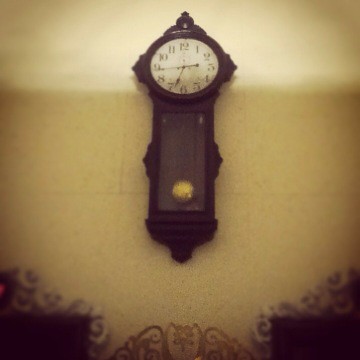This photograph, taken inside an old house, showcases a well-preserved vintage grandfather clock positioned against an off-white wall that appears weathered with age. The clock, crafted from rich wood, features a classic round clock face adorned with traditional numerals. Below the face, the wooden structure extends into a lengthy compartment, enclosed by a glass panel, revealing the long, metallic pendulum that rhythmically swings back and forth. The entire clock, encased in an elegant wooden frame, serves as a striking, nostalgic centerpiece within the room.